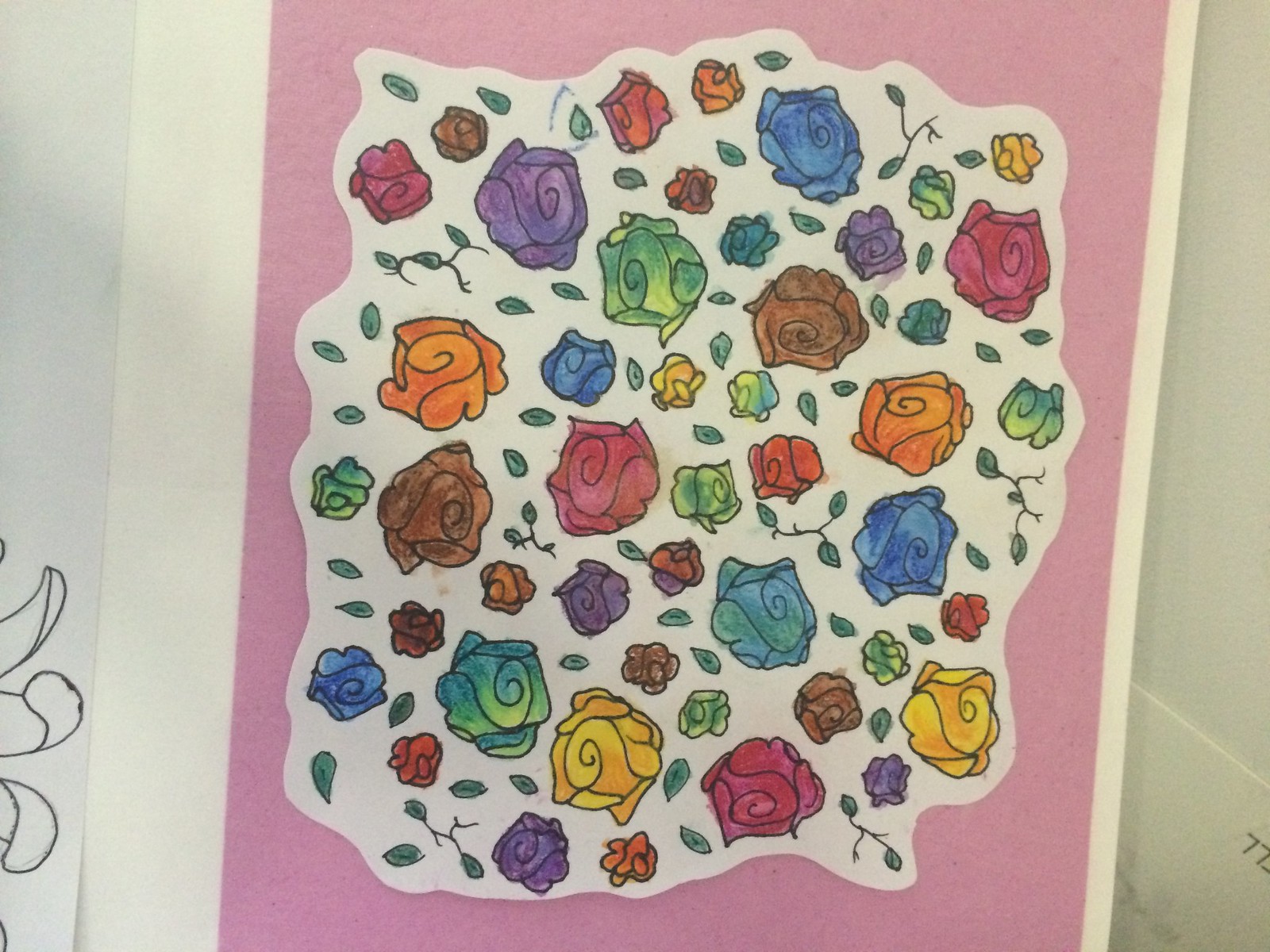This captivating photograph showcases a vibrant children's artwork, prominently displayed on a wall, which is likely within a home or a school setting. The image captures a vivid pink piece of construction paper serving as the backdrop for a smaller, white sheet of paper that has been creatively adorned with an array of roses. Each rose is meticulously outlined in black and infused with a spectrum of colors, portraying a unique individuality. The flowers vary in size, adding an intriguing depth and character to the composition. Interspersed among the blooms are delicate strings of leaves and standalone leaves, enhancing the organic feel of the piece. The photograph also hints at its context, with the edge of an adjacent drawing partially visible on the left, suggesting it is part of a larger collection of children's artworks proudly exhibited on the wall.